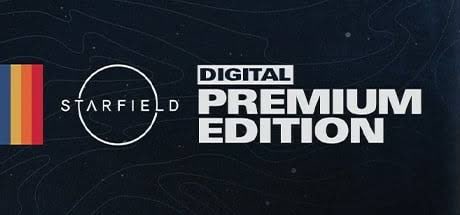This image is an advertisement for the game "Starfield," specifically showcasing the Digital Premium Edition. The logo features the word "Starfield" in white text, with a circular design that seamlessly integrates through the vertical lines of the 'T' and 'L' in "Starfield." Behind the text is a very faint contour map design in white lines set against a black background. To the left of the text, there are four stacked vertical bars in blue, yellow, orange, and red. The whole design is primarily monochromatic, except for these colorful bars, which add a striking contrast. The words "Digital Premium Edition" are prominently displayed in white, adding to the sleek and modern aesthetic of the advertisement.